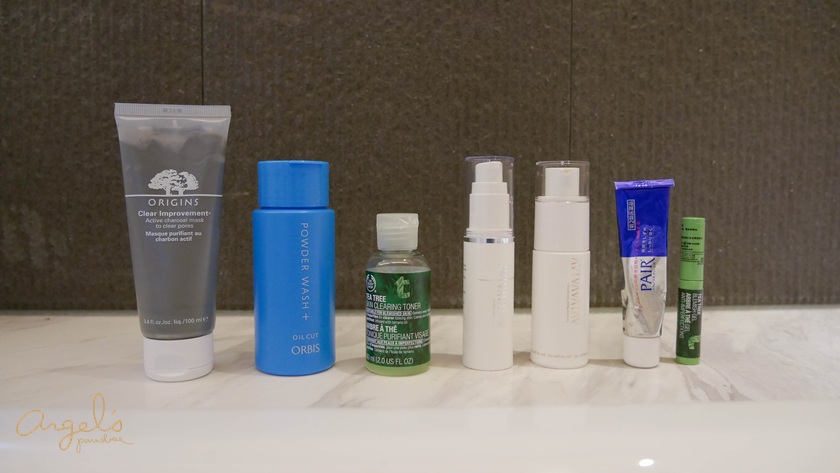The image captures a white countertop, possibly in a bathroom, with marbled accents toward the back that feature cream and gray hues. The backdrop consists of dark grayish-brown tiles with a textured surface. In the bottom left-hand corner, the word "angels" is visible, though the smaller word beneath it is not legible. The countertop is adorned with various skincare products. There is a gray tube with a white cap labeled "Origins Clear Improvement," a blue bottle labeled "Powder Wash," and a small, clear bottle with a green label that has unreadable text. Additionally, there is a white spray bottle with a cap, another white bottle with a spray mechanism and cap, and a tube labeled "Pear." Finally, there is a small, round green and black tube.